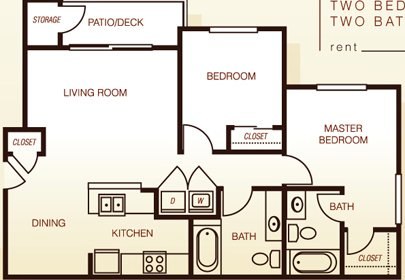This detailed blueprint of a two-bedroom, two-bath rental property, as noted in the upper right-hand corner where "two-bed, two-bath" is labeled with part of the "H" cut off, and "rent" written underneath, features a line drawing on a yellowish background with black lines. 

On the bottom left, the layout begins with the dining room, which is adjacent to the kitchen. The living room occupies the same width as the dining room and kitchen and is located directly above them. Between the dining room and living room, there is a closet. Above the living room, spanning the same width, is a space divided into roughly one-third storage area and one-third patio.

To the right of the dining room and kitchen (which share the same width as the living room), there is a bedroom situated next to the living room. Adjacent to the kitchen, there is a bathroom. Beyond this, towards the back, lies the master bedroom, which is about half the length of the other bedroom, as well as an additional bathroom. The two bathrooms are positioned next to each other, ensuring convenience. The master bedroom also contains doors leading to its exclusive bathroom and a closet, enhancing its functionality.